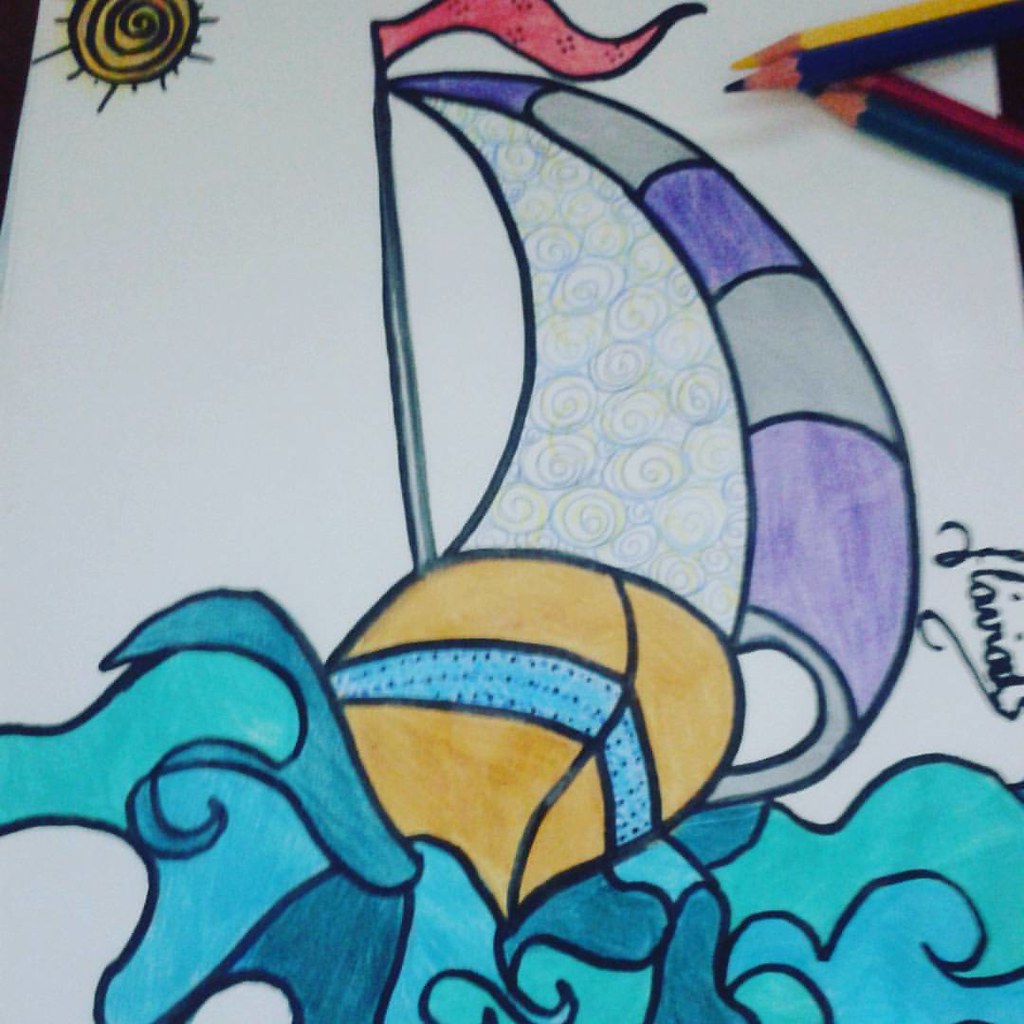This close-up image captures an intricately colored scene from a coloring page. The focal point is a boat navigating vibrant waves, each wave meticulously shaded in varying hues of blue. The boat itself features a bright yellow body accentuated by a light blue stripe. Its sail, adorned with purple and gray sections, showcases artistic swirls towards the back. Atop the sail, a red flag flutters on its pole. Adding to the picturesque scene, a spiral-shaped yellow sun radiates from the top left corner of the image. There is also a signature, penned in black, prominently located in the middle right of the page. In the top right section of the image, three colored pencils – yellow, blue, and red – lie neatly, perhaps tools of the artist's trade.